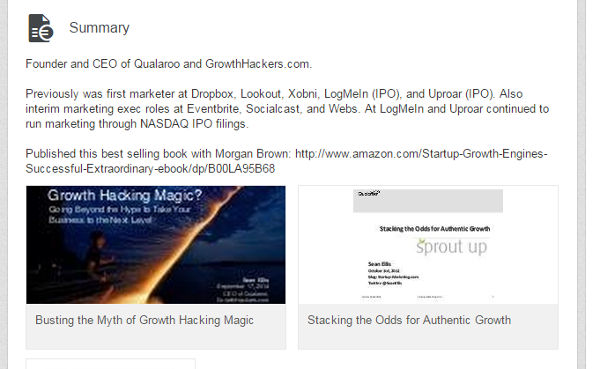Screenshot of a webpage displaying an article with a predominantly white background. At the top left, there's a title labeled "Summary" accompanied by a document icon. Just below this, it provides a brief professional biography indicating the individual is the Founder and CEO of Qualaroo and growthhackers.com. The text continues to list previous roles, such as being the first marketer at companies like Dropbox, Lookout, Zobree, Logmein (noted as IPO), and Uproar (also IPO). Additionally, it notes interim marketing executive roles at Eventbrite, Socialcast, and Webz, with a specific highlight on running marketing through NASDAQ IPO filings at Logmein and Uproar.

The summary also mentions the publication of a bestselling book co-authored with Morgan Brown, accompanied by a URL link to the book's Amazon page. Below this biographical section, the page features two articles side-by-side, each with an image at the top. The first article, titled "Busting the Myth of Growth Hacking Magic," is on the left, and the second article, titled "Stacking the Odds for Authentic Growth," is on the right.